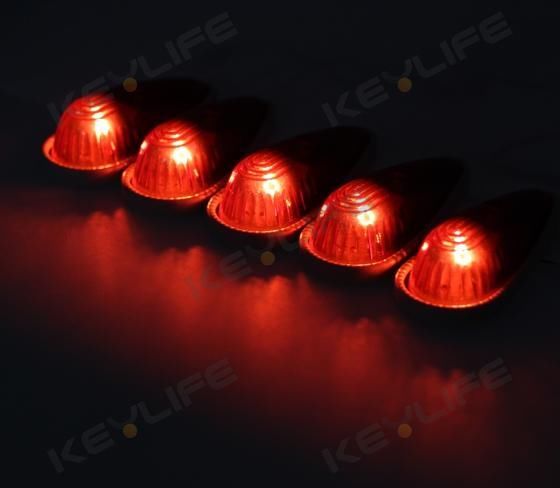In this color photograph, taken in an intensely dark environment, five equally spaced, illuminated red lights with bulbous plastic covers form the central focus, positioned diagonally from the bottom right up to the top third of the image. Each light features an overexposed bright white center, casting shadows beneath them and a curved, undulating reflection extending from the top left to the bottom right. The photo is heavily shadowed, obscuring any indication of what the lights are attached to or their purpose. The image is watermarked repeatedly with "KEVLIFE," with each "V" featuring a pale orange circle at the joining of its lines. The stark contrast of black and red in the background adds to the enigmatic and potentially futuristic feel of the lights, reminiscent of science-fiction cryosleep pods or a row of glowing firefighter helmets.